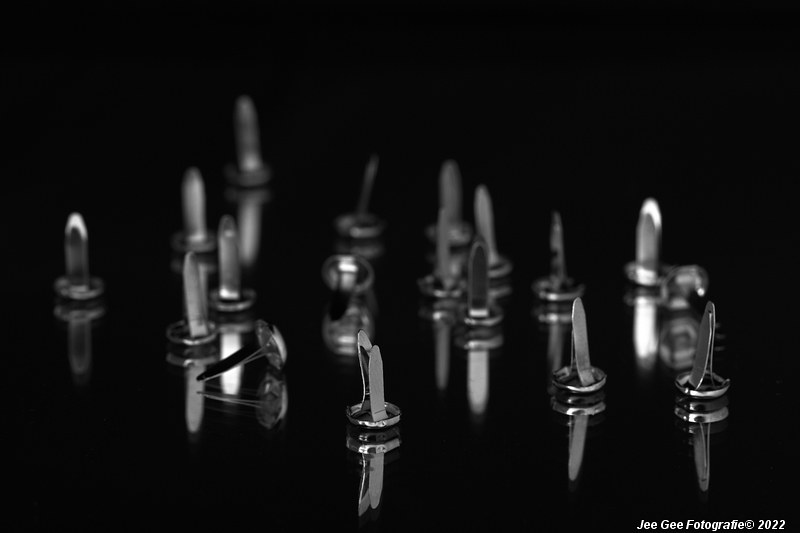This digital photograph features a set of silver fasteners used for securing notebook paper by flattening their metal flaps. The fasteners, with round discs at the base and two flared metal clips, are neatly aligned against a pitch-black background. The metallic sheen and uniform shape of the 10 or 11 fasteners are evident, with a few appearing slightly faded due to the image's depth of field. Most fasteners stand upright, while some lie on their sides, each reflecting off the shiny surface beneath them. In the bottom right corner, white text reads "GG Photography © 2022."